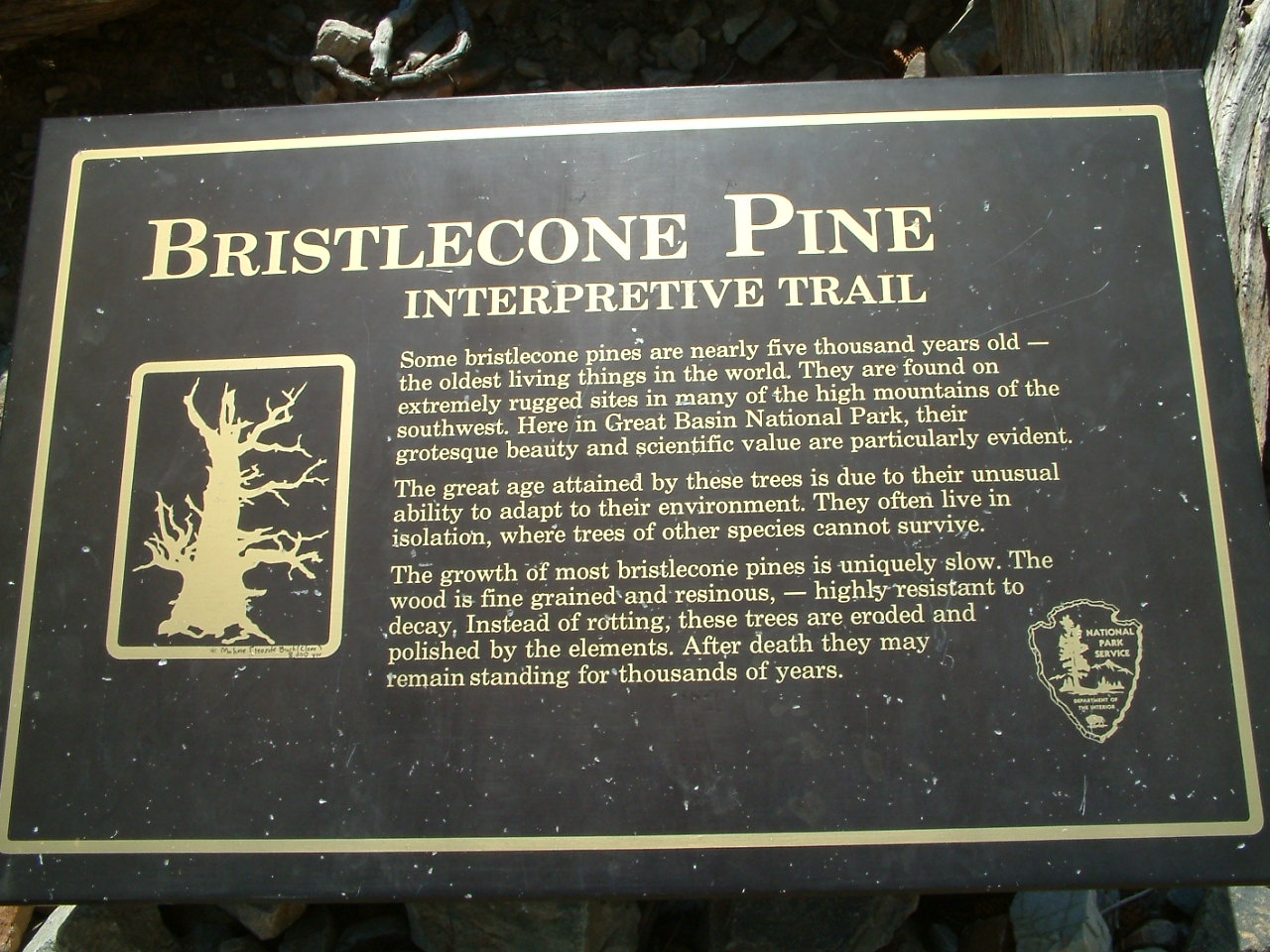This image depicts a detailed, photorealistic plaque located on a trail, framed by a gold, shining border against a black stone background flecked with white. The plaque is titled "BRISTLECONE PINE" in ornate, all-capital letters, followed by "Interpretive Trail" just below it in smaller text. Beneath the title, a comprehensive paragraph explains that some bristlecone pines are nearly 5,000 years old, making them the oldest living things in the world. These trees are native to extremely rugged sites in the high mountains of the southwest, including Great Basin National Park, where their grotesque beauty and scientific value are notably evident. The text elaborates on the trees' unique slow growth, fine-grained, resinous wood, and remarkable resistance to decay, contributing to their longevity even after death as they remain standing for thousands of years, eroded and polished by the elements. On the left side of the image is another gold box containing the outline of a uniquely shaped, leafless tree. The bottom right corner features a National Park Service emblem resembling an arrowhead with a tree inside it, also rendered in the same gold.